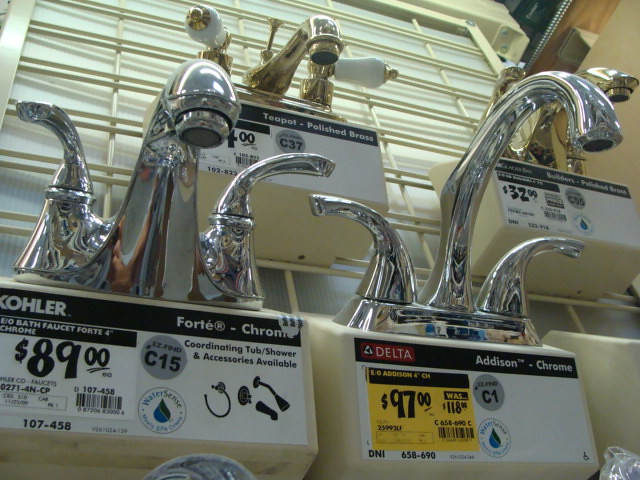The image captures a comical low-angle shot of four bathroom faucets displayed in a home improvement store, reminiscent of Home Depot or Lowe's. The unusual angle makes the faucets appear towering. From bottom left to top right, the faucets are: a Kohler Forte Chrome priced at $89 with matching tub and shower accessories; a Delta Addison Chrome on sale for $97, previously $118; a teapot-styled polished brass faucet with ornate white handles; and a Glacier Bay Builders-grade polished brass faucet priced at $32. The display includes brand names, prices, and model numbers, all neatly arranged on a frame shelving rack.